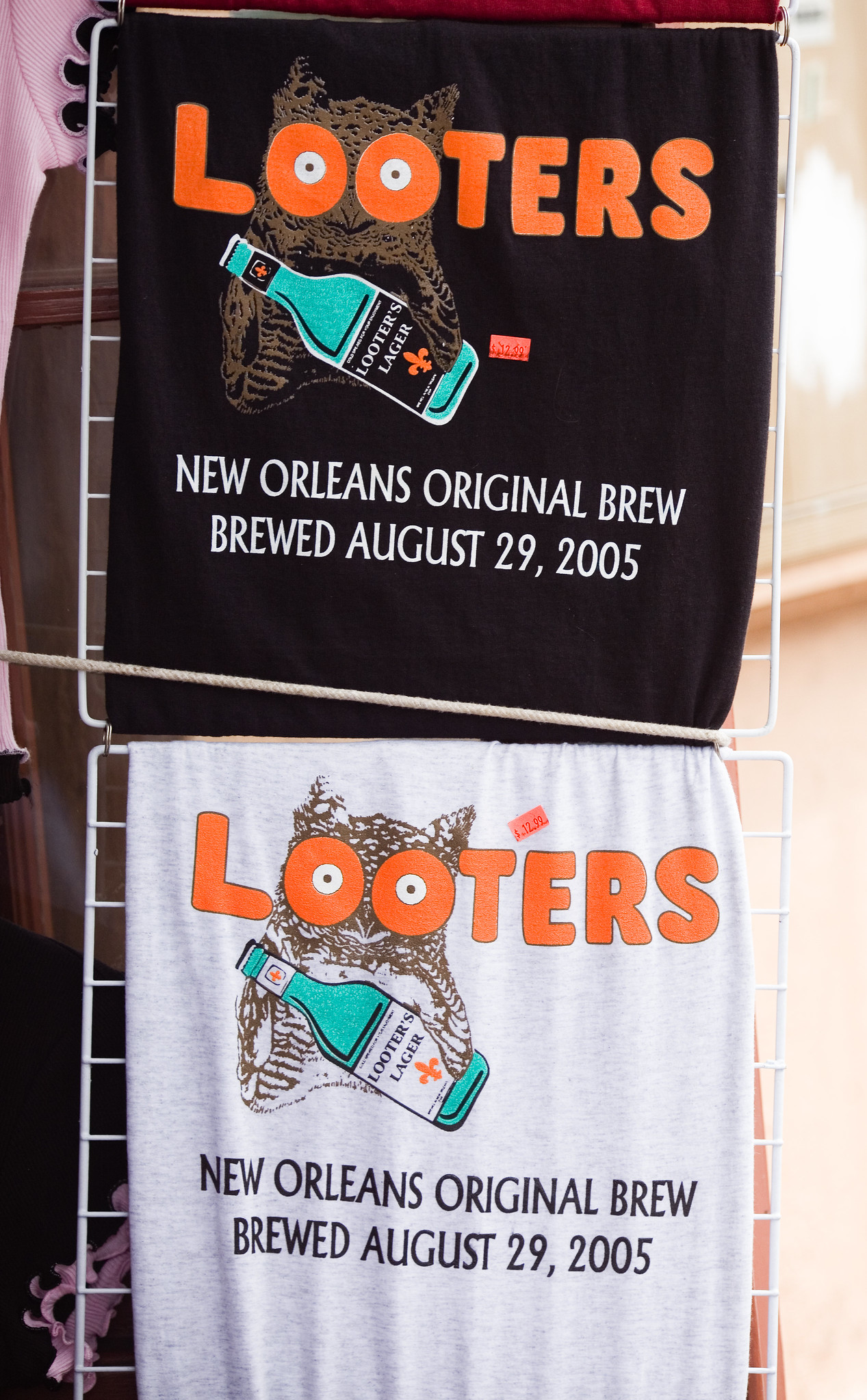The image displays two vertically-aligned, rectangular cloth banners—or possibly t-shirts—each featuring an advertisement for "Looters Lager" beer. Both banners hang from a white wire frame, with the top one having a black background and the bottom one having a white background. Each banner prominently displays the word "LOOTERS" in large orange letters, with the two O's designed to resemble eyes, and an owl peering through them. The owl is grasping a turquoise bottle of Looters Lager. Beneath the owl, the text reads "New Orleans original brew brewed August 29, 2005," with the text color contrasting against the respective background color. Additionally, a small red price tag indicating $12.99 is visible. The setting reveals a glimpse of another shirt in the background, along with a light-colored floor and wall.